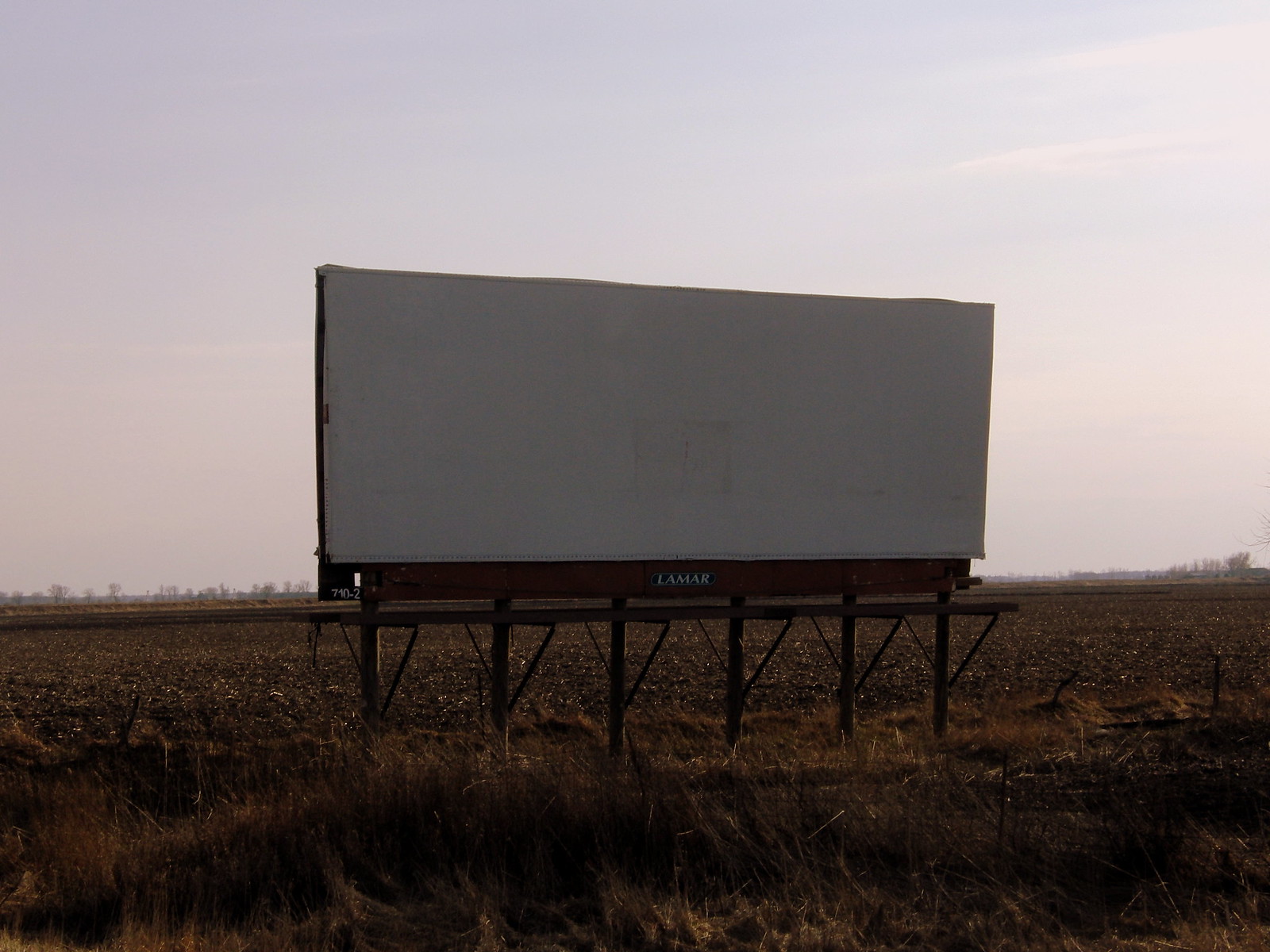In the photograph, a blank white billboard stands prominently in a vast, barren landscape, typical of West Texas. The billboard, marked with the "Lamar" logo in white on its brown frame, sits elevated on six wooden posts. Its surface shows signs of weathering, with the white paint slightly peeling and dirty in places. The surrounding ground is a mix of brown tilled soil and patches of dry, dead grass, indicative of a recently harvested cotton field, with leftover flecks of cotton visible. In the far background, sparse, leafless trees dot the flat horizon, aligning roughly two-fifths of the way up the image. The sky above is a light gray-blue, strewn with wispy white clouds that lend a hazy appearance to the horizon, emphasizing the desolate and bleak nature of the scene.